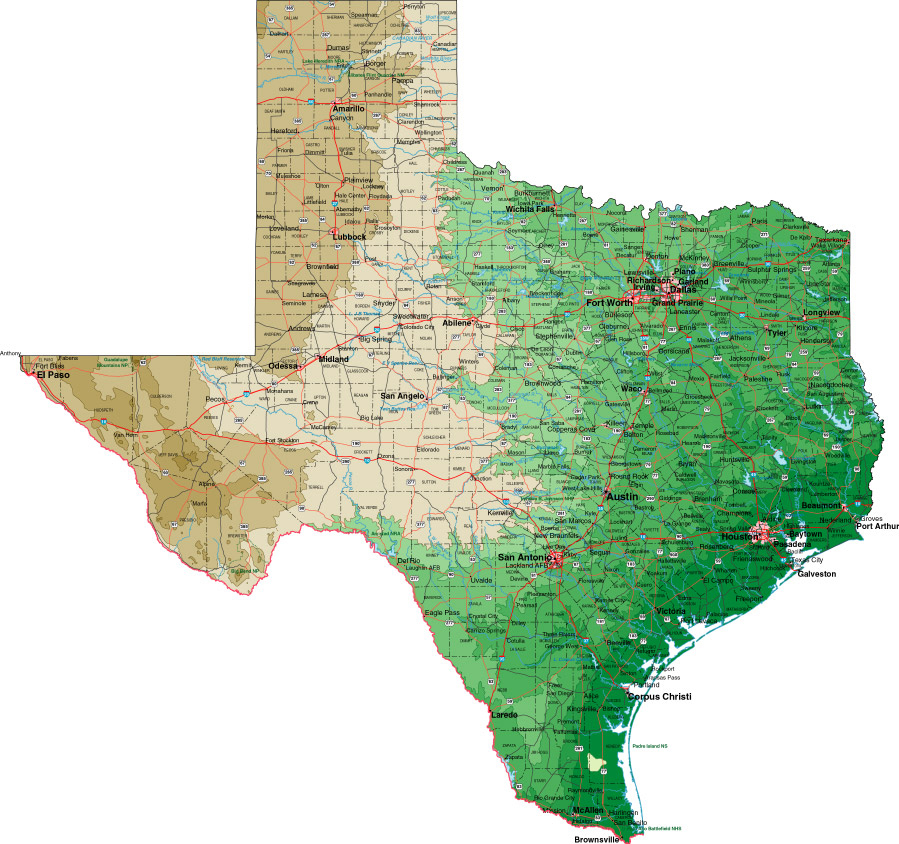This image is a detailed topographical map of Texas, illustrating the state's diverse terrain and climatic zones. The map is divided into three distinct color-coded regions: the left portion of the state is depicted in a darker brown shade, indicating arid and desert-like areas, particularly around the cities of Amarillo, Lubbock, Odessa, and El Paso. Moving towards the center, the map transitions into a lighter beige color around towns such as San Angelo, Midland, and Abilene, signifying semi-arid zones. The right-hand side and the southern part of the map are predominantly green, representing forested and grassy areas that receive more rainfall. This green region covers nearly half the state. The map also features numerous roads, towns, cities, lakes, and rivers, although most of these details are too small to read clearly.